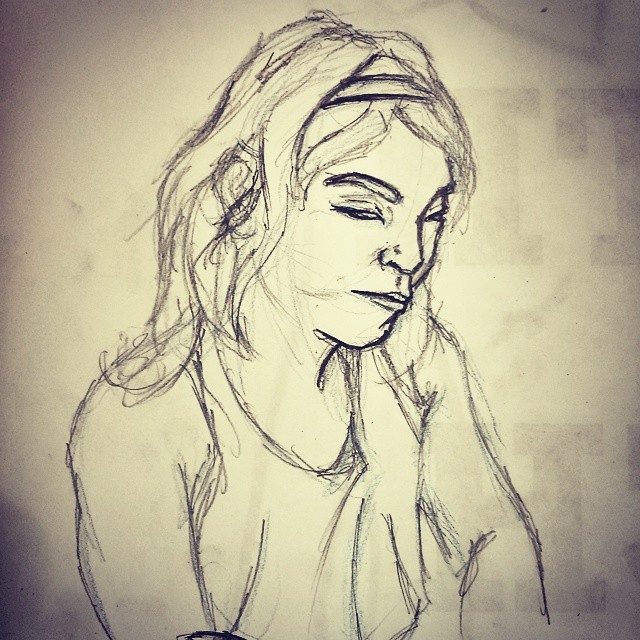This is a detailed pencil sketch of a woman with shoulder-length hair, which appears slightly tangled and unruly, particularly on one side. She wears a headband that partially tames her thick locks, although some stray strands cross her face. Her eyebrows are thick and bushy, adding a strong frame to her partially closed eyes. She has a sharply defined nose, and her lips rest in a neutral expression. Her well-defined philtrum (the indent above her lip) is accentuated with darker shading. The woman is dressed in a loose, baggy shirt that bears some stray pencil markings, especially around the sleeves. The white paper that forms the background exhibits hints of faded, stamped letters, adding an element of texture and depth to the sketch.